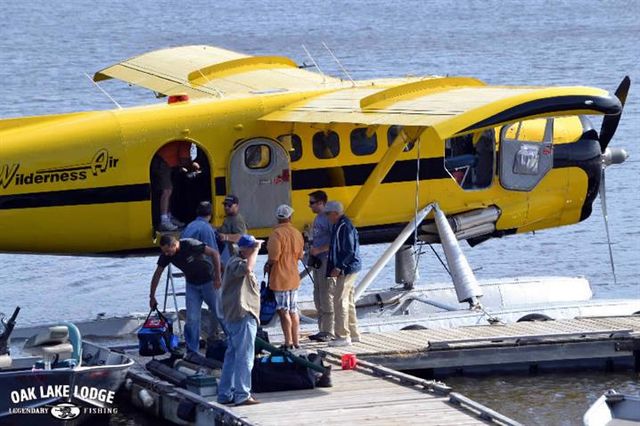In the photograph, a vibrant yellow seaplane with black trim is prominently featured, docked beside a calm lake. The plane, clearly branded as "Wilderness Air," has an open door and four visible windows along its side. The propeller at the front is stationary. The underside and part of the plane's side are accented with black. Around eight people are gathered on the wooden dock, some appearing to be boarding the plane while others, possibly workers, assist. A man inside the plane is visible, dressed in a yellow and orange top with dark green shorts, sneakers, and white socks. Near the dock, to the left, there is a small boat with "Oak Lake Lodge" inscribed in large white capital letters, hinting that the seaplane services this lodge renowned for its legendary fishing. The overall scene suggests it's daytime, with the water notably calm, enhancing the serene backdrop.